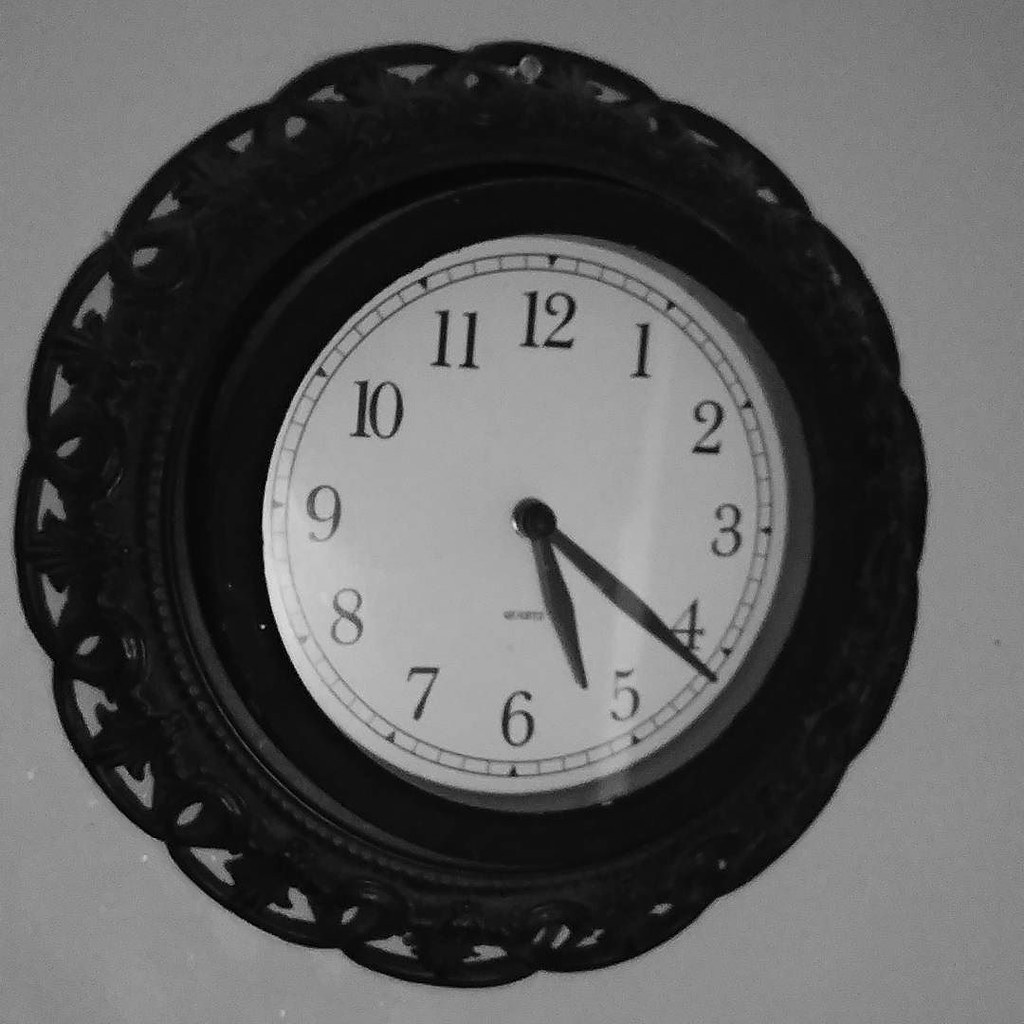A detailed description of a clock:

The image showcases a wall-mounted clock, viewed from an angle that makes it appear slightly off-center. The clock features a clean, white face contrasted by solid black hands and large, bold numerals for easy readability. It is encased in a round black support that seamlessly connects to a decorative outer ring. This outer ring is scalloped, creating a pattern through which the gray wall it is mounted on is visible. The clock displays the time as 5:21. The detailed craftsmanship and classic color palette give the clock an elegant yet functional presence on the otherwise understated gray wall.